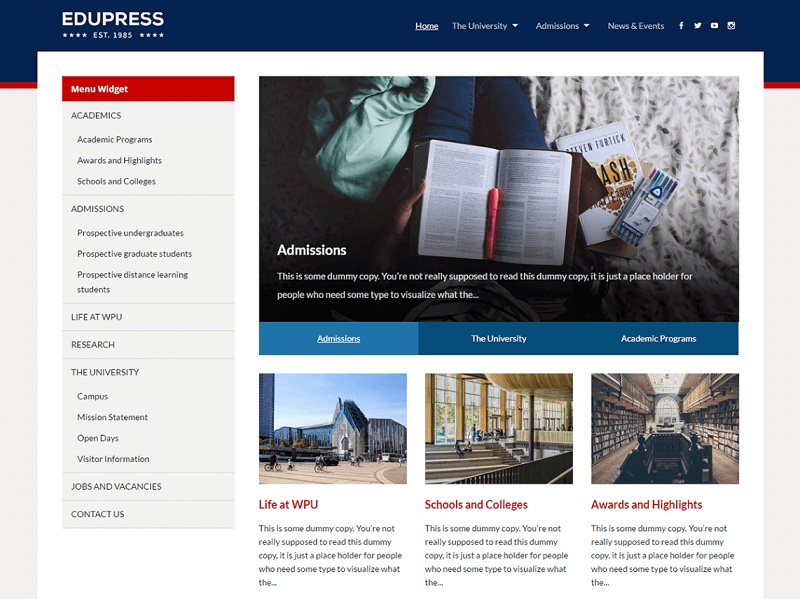Screenshot of the EduPress Website Interface

This detailed webpage screenshot showcases the interface of EduPress, a website established in 1985. At the top of the screen, the website's header is displayed, featuring the EduPress logo followed by four small stars, emphasizing its long-standing reputation. The header title and menu options are rendered in white text on a navy blue background, creating a sleek and professional look.

The primary navigation menu includes:
1. **Home** (underlined, indicating the current page)
2. **University** with a drop-down arrow hinting at additional sub-menu items
3. **Admissions** with a drop-down arrow
4. **News and Events**

On the left side of the page, there is a prominent sidebar featuring various navigational options. The sidebar categories are colored in light black text on a white background, except for "Menu Widget," which is highlighted with a red background. The sidebar sections are as follows:

- **Academics** (in capital letters)
  - Academic Programs
  - Awards and Highlights
  - Schools and Colleges
  
- **Admissions** (in capital letters)
  - Prospective Undergraduates
  - Prospective Graduate Students
  - Prospective Distance Learning Students
  
- **Life at WPU** (in capital letters)

- **Research** (in capital letters)

- **The University** (in capital letters)
  - Campus
  - Mission Statement
  - Open Days
  - Visitor Information
  
- **Jobs and Vacancies** (in capital letters)

- **Contact Us**

To the right section of the webpage, there is a highlighted rectangle labeled "Admissions," followed by a dropdown menu with other quick-access options:
- **Admissions**
- **The University**
- **Academic Programs**

Additionally, three square boxes are present, each containing brief descriptive sentences:
1. **Life at WPU**
2. **Schools and Colleges**
3. **Awards and Highlights**

This structured and visually appealing layout provides users with intuitive navigation options to explore various aspects of the university and its offerings.